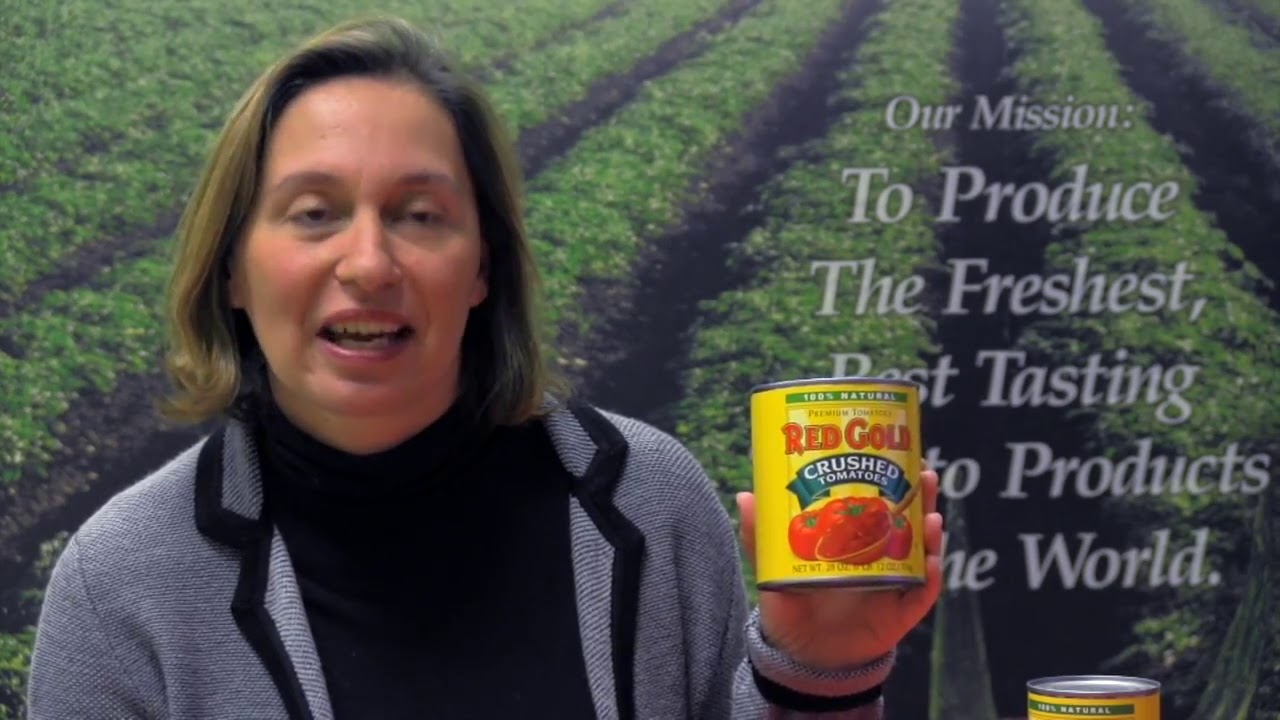A woman with short brown and blonde hair, wearing a gray sweater over a black shirt, holds up a can of Red Gold crushed tomatoes. The can, featuring a bright yellow label with images of tomatoes and text stating "100% natural" and "premium tomatoes," prominently displays the Red Gold brand in red and gold letters. Her mouth is slightly open as if she is speaking, and her eyes are partially closed. In the background, a mission statement reads, "Our mission to produce the freshest, best tasting tomato products in the world," with fields of tomato plants visible behind her. Another, smaller can of a similar product is also present in the image, which has the appearance of a nostalgic frame from a vintage commercial, possibly from the 80s or 90s.